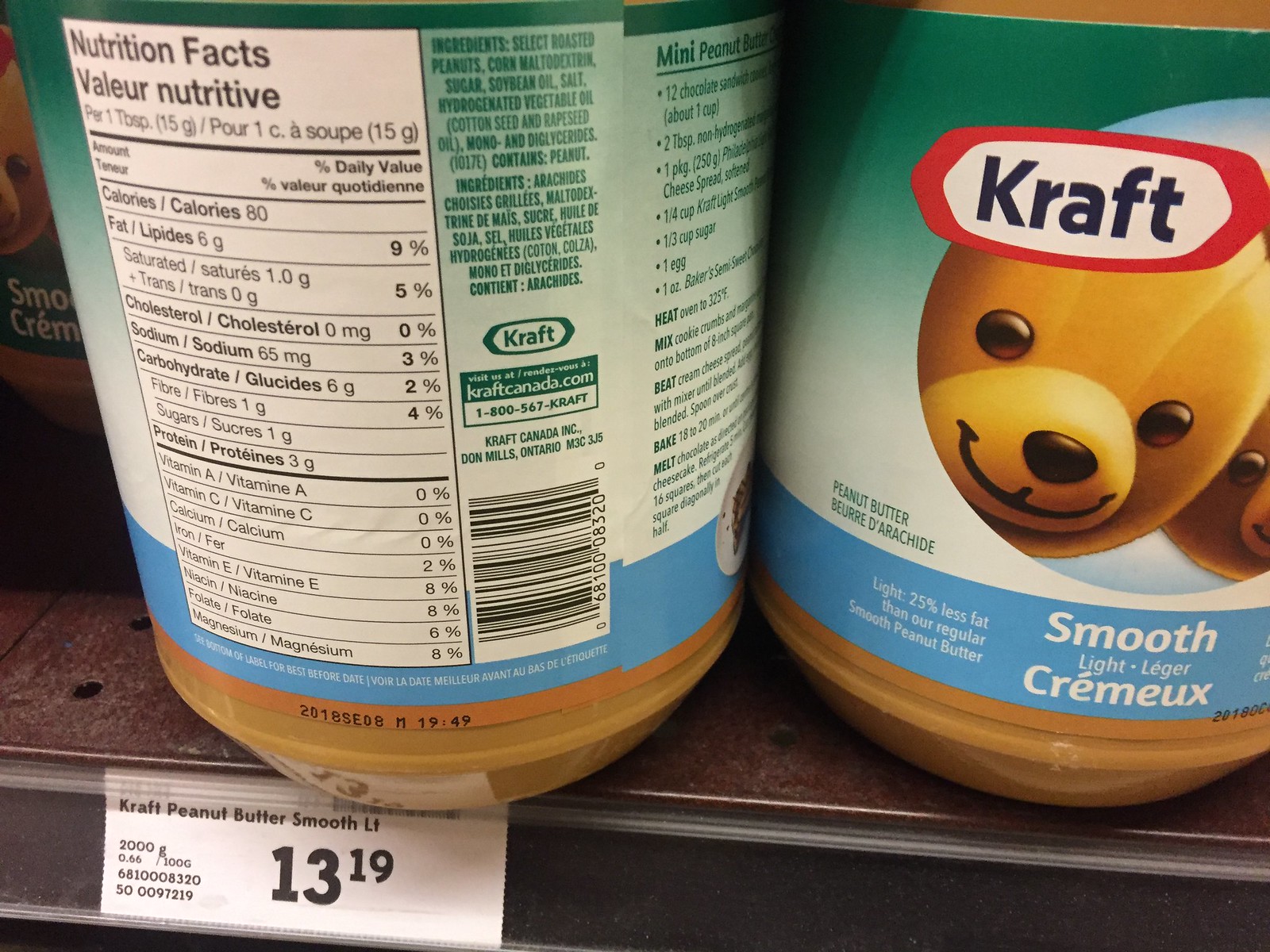This detailed photograph captures a well-organized shelf displaying priced jars of Kraft Smooth Peanut Butter. The price tag prominently reads $13.19. There are three jars of peanut butter, although the third jar is only partially visible. Among the two jars in full view, the jar on the left reveals the nutrition facts labeled in both English and French as "Nutrition Facts" and "Valeur Nutritive." This label presents a green to light green gradient background, complemented by a light blue banner at the bottom. The jar on the right showcases the front label, featuring the iconic Kraft logo encircled in red. Displayed on this label are two teddy bears smiling at the camera. Beneath the bears, it states, "Smooth Peanut Butter Light," noting that it contains 25% less fat than the regular smooth variety.